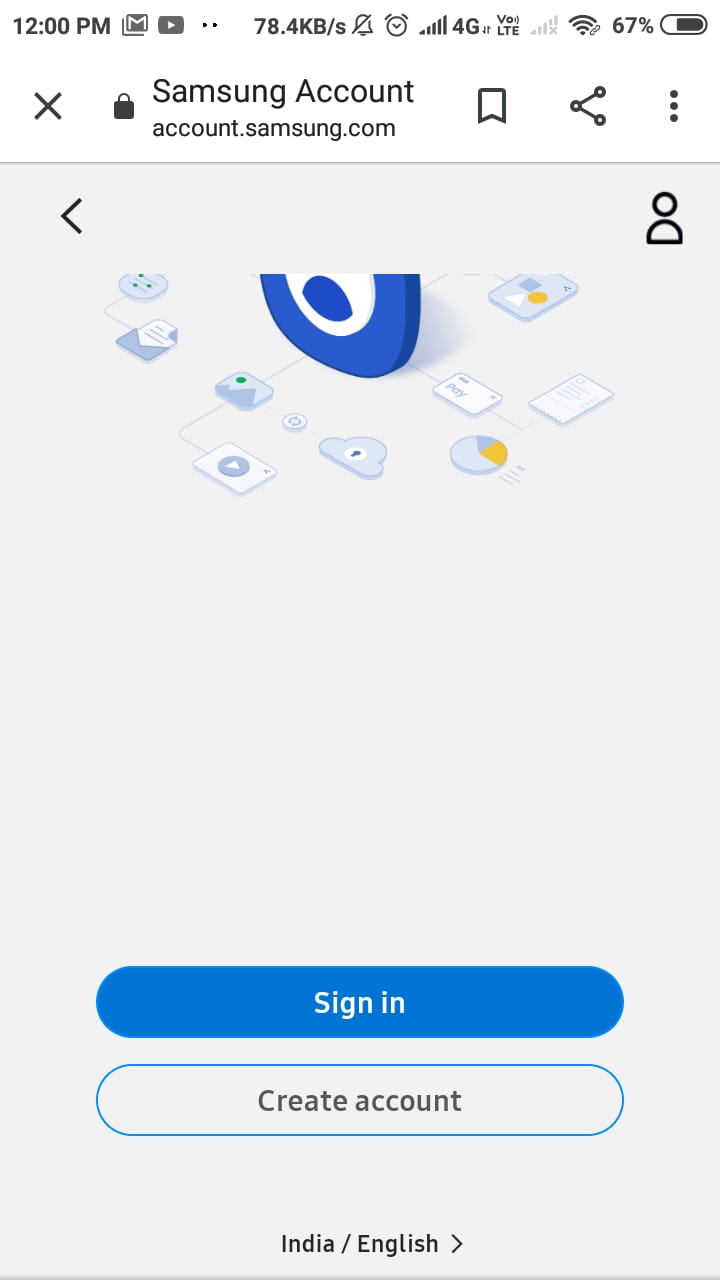This image is a detailed screenshot from a smartphone, featuring a user interface for a Samsung account. The header section of the screen is white, with very dark gray fonts for better readability. On the upper left, the time is displayed as 12 p.m. On the upper right, the status bar shows the battery level at 67%, alongside icons for Wi-Fi and the 4G network. 

Centered beneath the header is the text "Samsung account," followed by the web address "account.samsung.com." To the left of this text is an 'X' icon, and on the right, there are three additional icons: a save icon, a connected three-dots icon, and a vertical three-dots menu icon.

The background color of the main section is a very light gray. At the top, there is a graphical element featuring a partially visible blue circle, enclosing a white circle and another smaller blue circle within it. Below this graphic, a blue, rounded rectangle button with the white text "Sign in" is prominently displayed. Beneath this button is another outlined button with the text "Create account," which is gray with a blue outline matching the background color.

At the very bottom of the screen, the text "India / English" is displayed, next to a right-pointing triangle, likely indicating a language or region selection option.